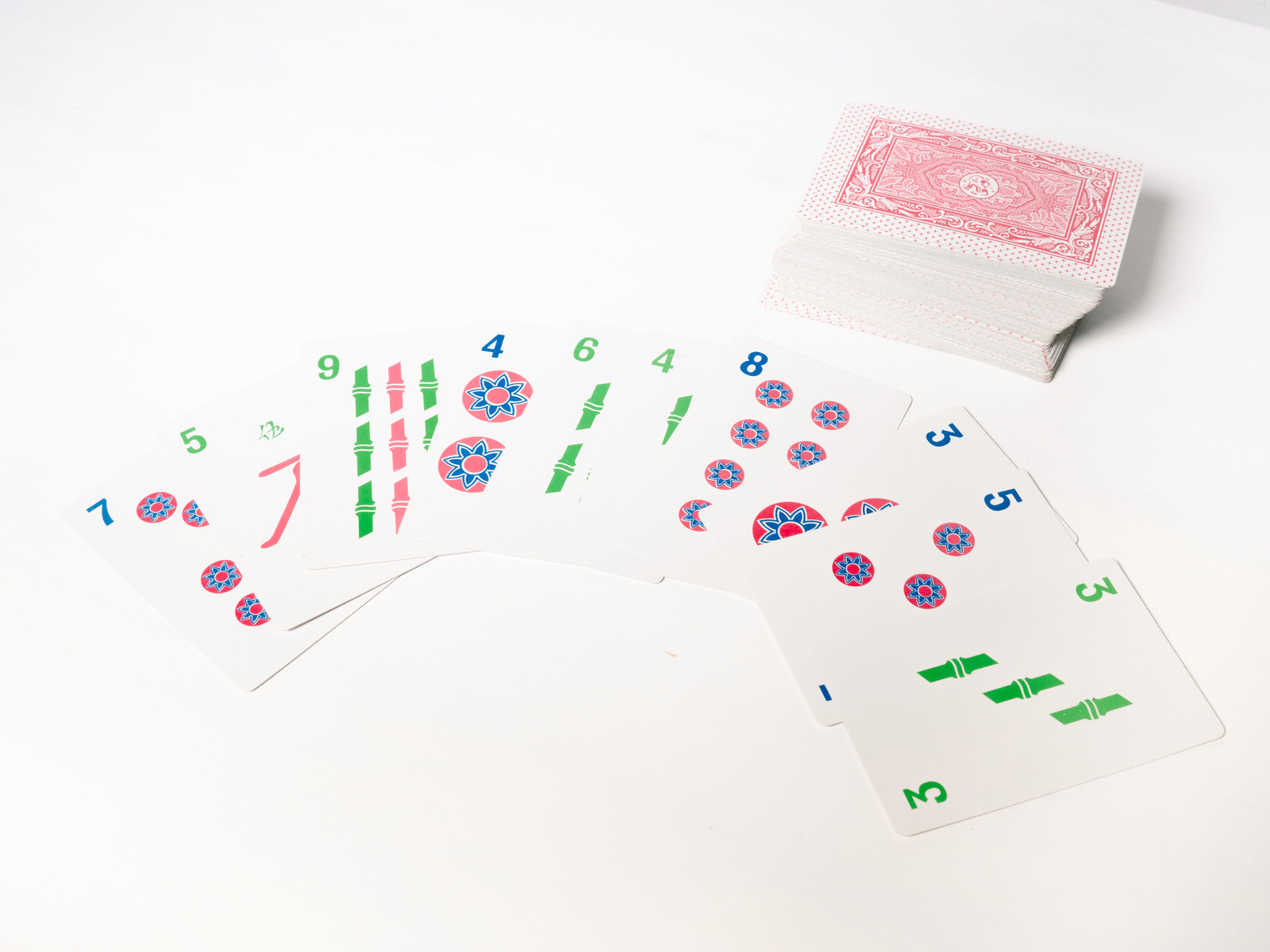A landscape-style photo features a deck of cards placed on a white table. In the top right corner, there is a neatly stacked pile of cards, with the card on top displaying its intricate red and white back design, adorned with fine line patterns. In the foreground, ten cards are laid out in a row, each showcasing a different number and color. The leftmost card shows the number 7, with four circles outlined in red and filled in blue. Next to it is a card with a green number 5. Following in sequence are a green number 9, a blue number 4, a green number 6, another green number 4, a blue number 8, a blue number 3, a blue number 5, and finally, a green number 3. The white table provides a clean and simple background, highlighting the vivid colors and distinct designs of each card.